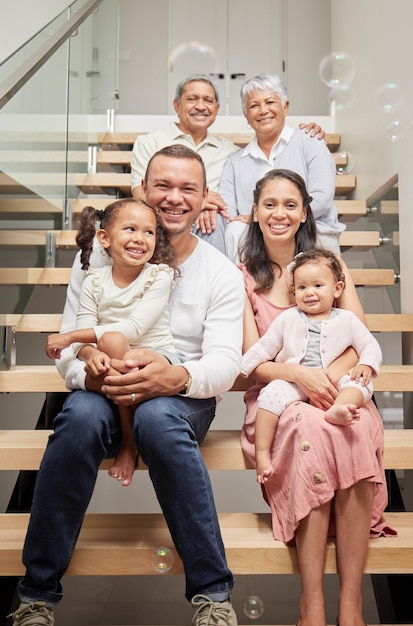In a warmly lit family photo, six individuals are seated on a light brown wooden staircase adorned with a modern glass railing to the left and a metallic handrail. The background features off-white walls and a double door with black handles at the top of the stairs. Bubbles float whimsically throughout the image, adding a playful atmosphere. 

At the top of the stairs sits an older man and woman; the man gently rests his arm on the woman's shoulder. He is dressed in a light mint green shirt, while she wears a light gray top. In front of them sits a younger couple: the man, wearing a white long-sleeve shirt and blue jeans, and the woman, dressed in a pink dress. Each parent holds a child on their lap. The man cradles a girl, around four to five years old with brown hair in pigtails, who gazes off to the side. The woman holds a younger girl, possibly one to two years old, adorned in a very light pink sweater and capris. Both children are barefoot.

Everyone in the image wears cheerful expressions, capturing a moment of familial joy amidst the light-filled surroundings.